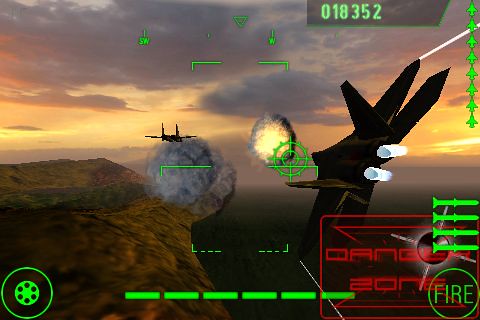The image depicts a vibrant computer game screen showcasing an aerial combat scenario. The top of the screen features a score displayed against a gray background in bright green digits, reading "018352." Along the right side of the screen, green airplane icons are vertically aligned. Just beneath these icons are small green missile images arranged in a circle, indicating four available missiles. At the bottom of the screen, the word "FIRE" is boldly written in uppercase green letters. On the bottom left-hand corner, there is another circular graphical element with a smaller circle inside and tiny holes around its edges, simulating a targeting reticle.

In the main gameplay area, the viewer can see a fighter jet flying sideways, with another aircraft visible ahead of it. The sky is adorned with scattered clouds and a setting sun, providing a dramatic backdrop. The foreground includes several gray spears and, to the left, a cliff with a grassy surface, adding depth and detail to the environment. The overall scene captures the intensity and detailed elements of the aerial dogfight within the game.